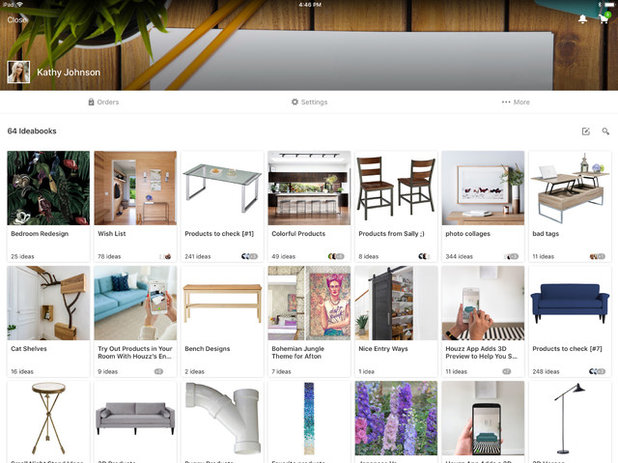The image showcases the profile page of Cathy Johnson on a furniture retailer's website. At the top, there is a banner image featuring a wooden fence adorned with a plant, providing a rustic backdrop. In the foreground, a computer screen appears, displaying Cathy's profile picture to the left. Below her name, the page lists her "ideabooks," which are collections of various furniture items and decor pieces.

The content is meticulously arranged, featuring a diverse array of home furnishings and accessories. Prominently displayed are beds with accompanying trays, various styles of couches and side tables, as well as some plumbing equipment such as large PVC pipes. Artwork pieces are interspersed throughout, adding an aesthetic touch to her curated collections. 

Unique items like a lamp positioned in the lower right-hand corner catch the eye, and floral arrangements are exhibited in one of the bottom images. A picture of her iPhone, displaying a green-themed website, is also part of the collection.

Despite the detailed visuals, there is no immediately visible contact information, potentially relegated to fine print. Settings and other options are available, possibly comprising more information or configurations. The layout presents Cathy Johnson’s diverse taste in home furnishings and her enthusiasm for curating a broad spectrum of household items.